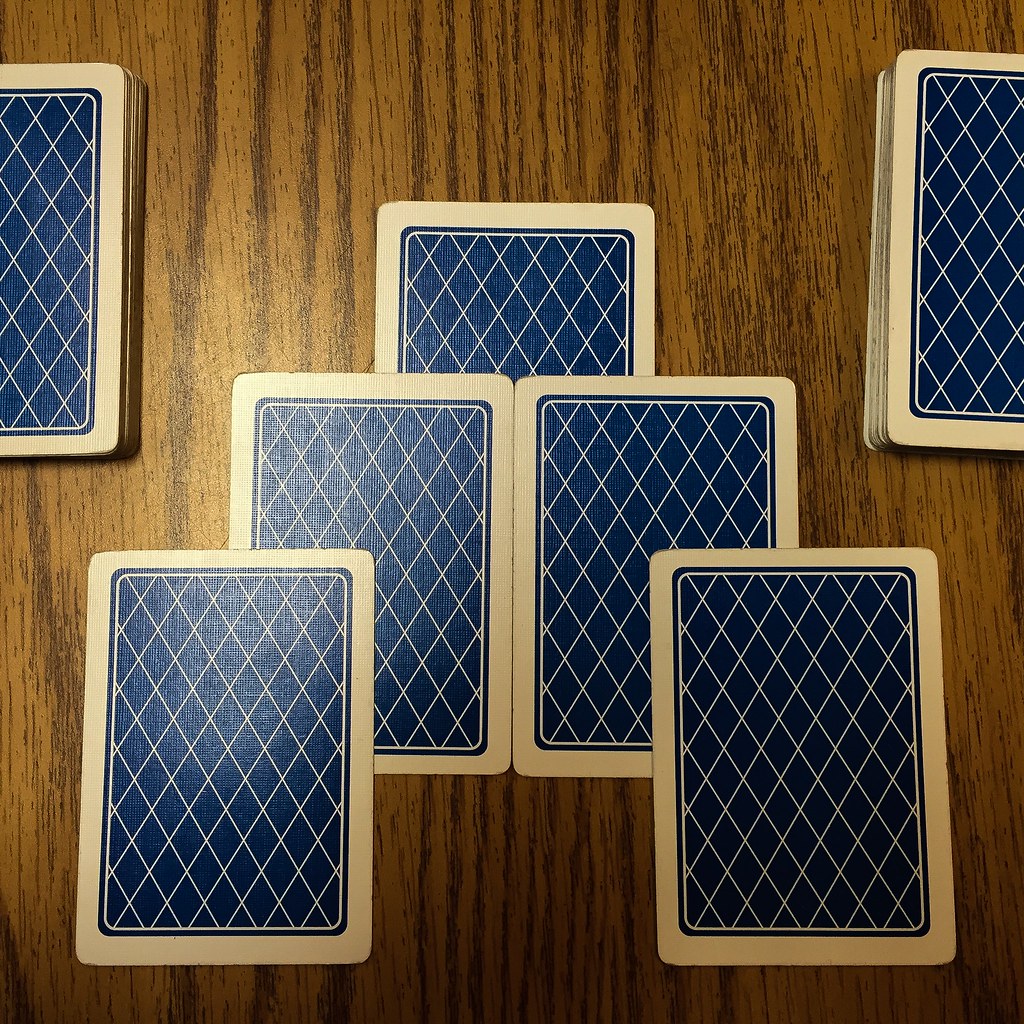This image captures a scattered arrangement of playing cards. In the upper right quadrant, a nearly half-deck stack of cards stands slightly off-center. Similarly, in the upper left, another almost half-deck stack is visible. The center of the image features five cards arranged in a layered formation: a single card lies flat in the middle, partly covered by two cards placed on top, with their top two-thirds visible. Over these, two more cards are positioned toward the right and slightly lower, allowing most of the second layer to be seen.

All the cards rest on a brown wooden tabletop, characterized by noticeable dark wood grain. The card backs display a distinct design: a white border encircles the edge, followed by a blue border, and then an intricate pattern of blue diamonds outlined in white. The white portions of the cards are visibly smudged and stained, suggesting extensive use over time.